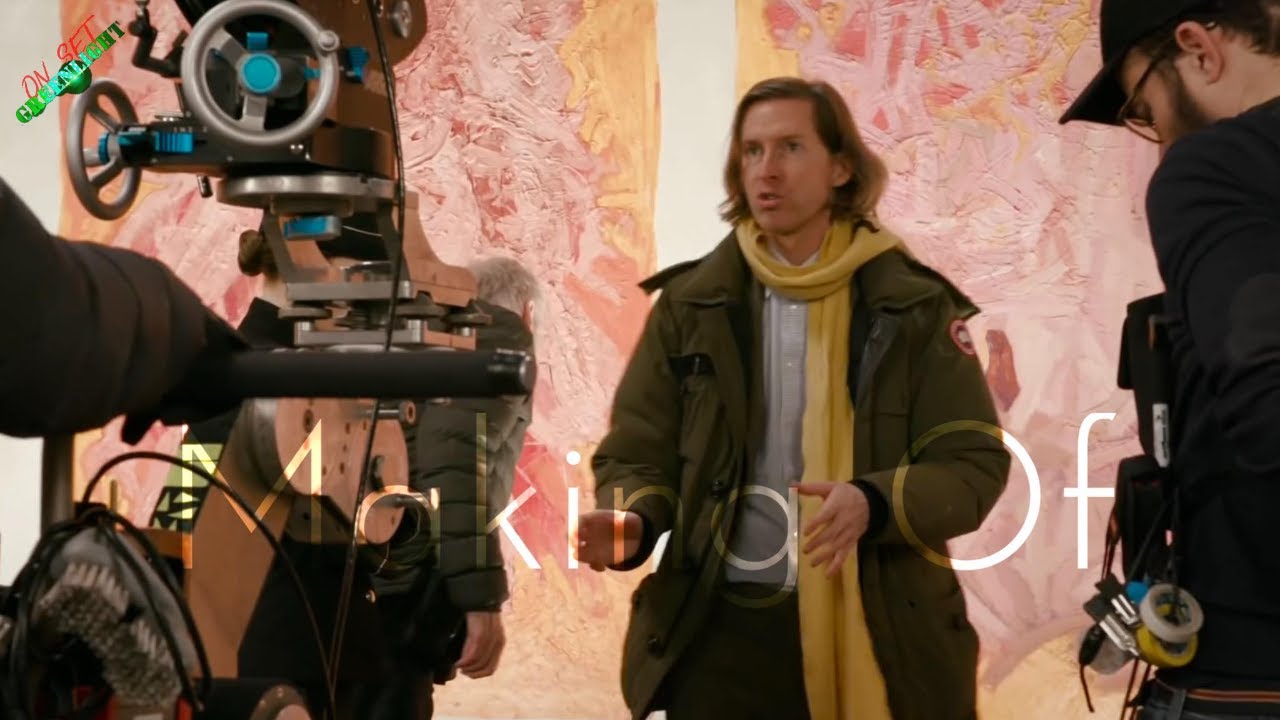This horizontally oriented photograph captures an indoor setting, featuring a man standing on a stage or set. Behind him, there's a distinctive pink backdrop with a white center, prominently displaying white text that reads "Making of." In the top left corner, there is more text in blue and red that says "on set." The man appears to be either a director or the main speaker, positioned centrally and mid-sentence, gesturing with his hands as if explaining or describing something. He is dressed in a green military-style jacket, a long yellow scarf, a dark gray undershirt, and slacks. He has long brown hair. Flanking him on both sides are members of a film crew. To his left, there's a large film camera apparatus, and to his right, another crew member, wearing a hat and glasses, is holding a device. The set behind him is somewhat blurry but includes varying shades of pink and some white and light green elements. The overall scene suggests a behind-the-scenes look at a film or commercial production.